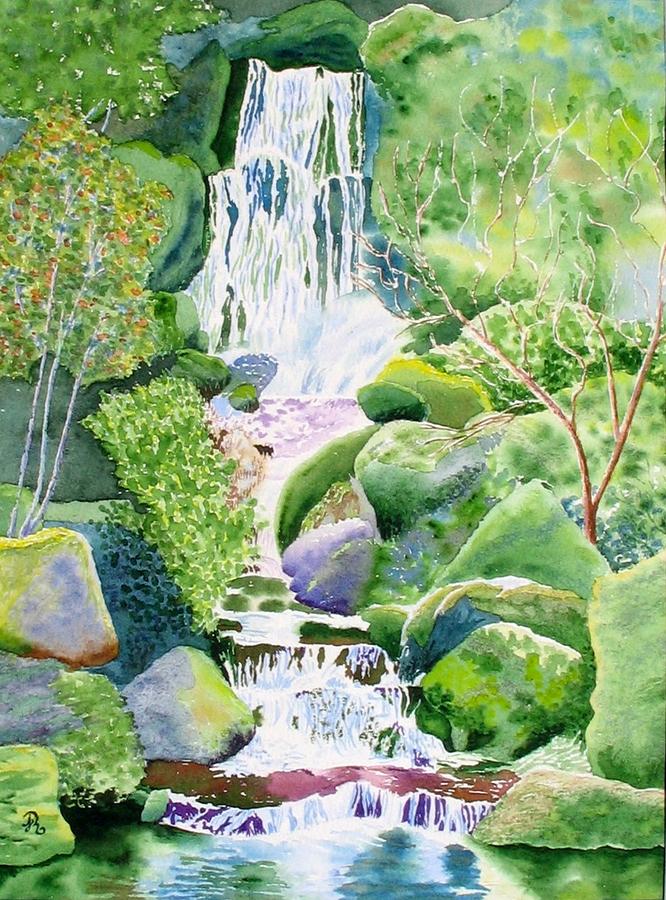This image depicts a watercolor painting of a lush, green landscape featuring a cascading waterfall at its center. The waterfall flows downward through multiple levels, surrounded by moss-covered rocks and a dense assortment of vegetation, including trees and bushes. Predominantly rendered in shades of green, the painting also incorporates accents of blue, purple, and hints of brown for the tree trunks. The water itself shimmers with light pastel hues of blue and purple, creating a dreamy, somewhat fantastical atmosphere. The entire scene is framed within a portrait-oriented composition and captures a sense of movement in the stillness of the painting. The artist has signed the piece with the initials "S.R." in the bottom left corner.